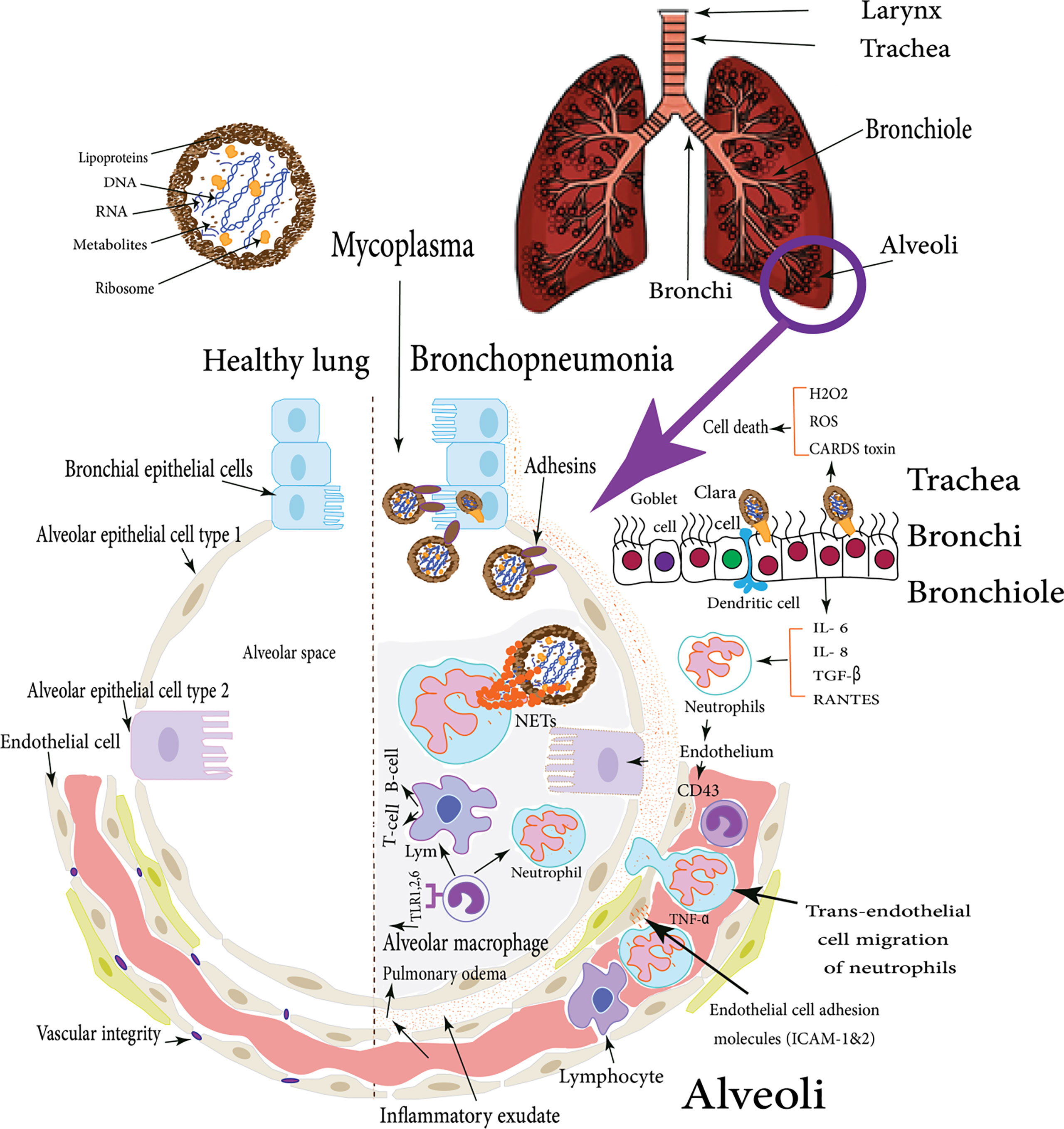This is a highly detailed scientific diagram, likely extracted from a biology textbook or medical website, illustrating the structure of the alveoli within the lungs. The image features a small depiction of human lungs in the top section, labeled with key structures such as the larynx, trachea, bronchi, bronchioles, and alveoli. A large arrow points from this depiction to a magnified, intricate diagram showcasing the alveolar structures.

In the center of the diagram is a dense network of arrows and labels, vividly colored in pink, purple, blue, red, green, yellow, and light brown. A dashed line in the middle separates the image into two sections. The left side, marked as "healthy lung," displays components like bronchial epithelial cells, alveolar epithelial cells, and endothelial cells in their normal state. 

Conversely, the right side, labeled "bronchopneumonia," illustrates the affected lung with additional elements such as lymphocytes, inflammatory exudate, alveolar macrophages, neutrophils, and more. Further labels detail the alveolar space, vascular integrity, adhesins, and nets, among other structures.

Numerous specific parts within the alveoli are labeled, including alveolar epithelial cell types 1 and 2, and other microscopic elements like lipoproteins, DNA, RNA, metabolites, and ribosomes, explaining the cellular makeup. The use of arrows and numerical callouts enhances the clarity and educational value of this medical illustration.